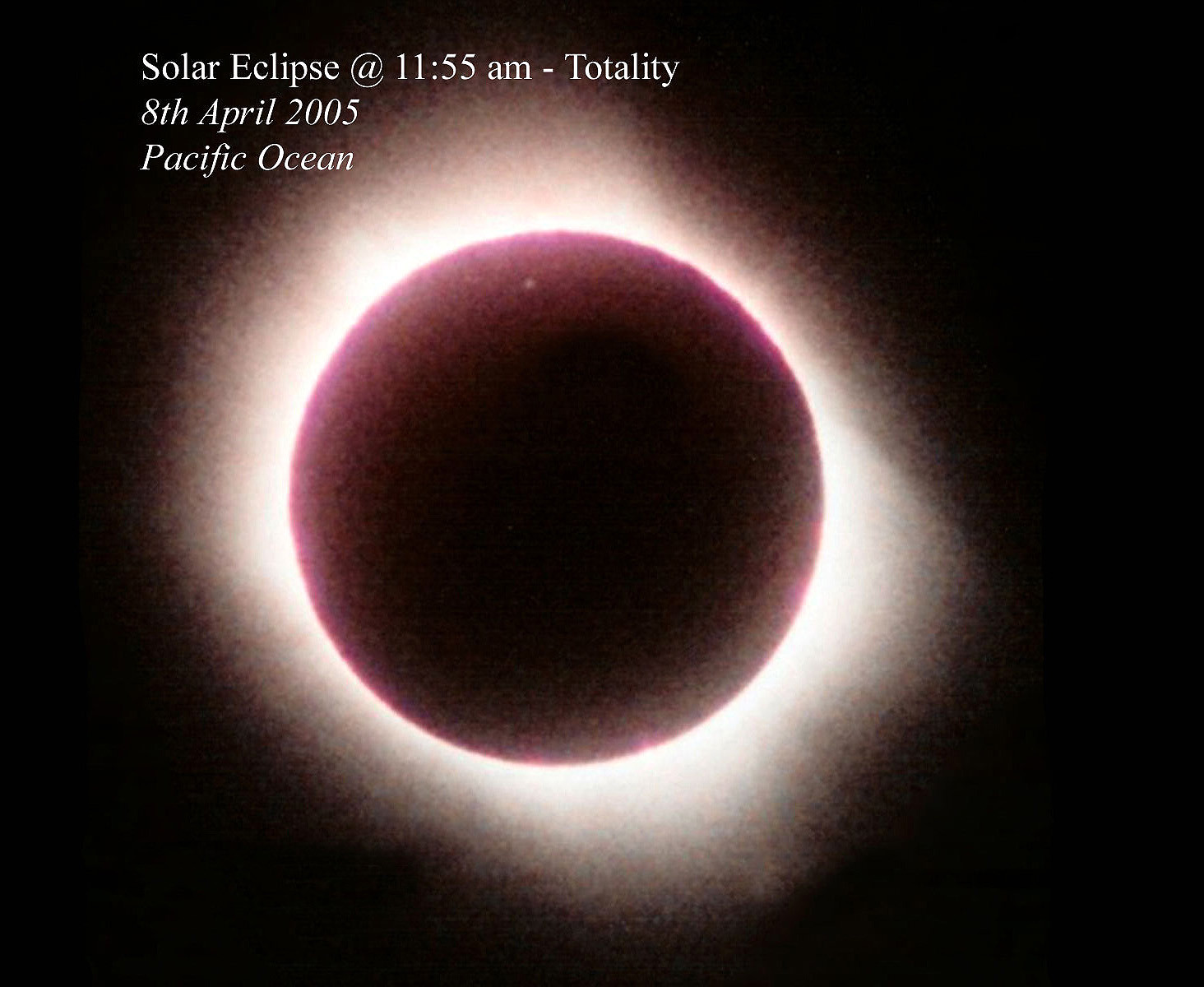The image depicts a striking solar eclipse against a completely black background. Central to the image is the full moon, creating an awe-inspiring sight as it fully blocks out the sun, resulting in a luminous halo—the corona—encircling its silhouette. The edges of the moon exhibit a reddish-pink hue, offering a stark contrast to its otherwise darkened, black core. The brilliance of the sun’s corona, though uneven and more pronounced on the lower side, creates an ethereal glow around the moon, further accentuating its celestial beauty. In the top left corner of the image, white text reads: "Solar Eclipse at 11:55 a.m. - Totality, 8th April 2005," followed by "Pacific Ocean." A small white speck is noticeable near the top of the moon, adding to the intricate details captured in this mesmerizing photograph. The notable graininess of the image lends it an authentic and raw essence, emulating the fleeting moment of cosmic alignment.